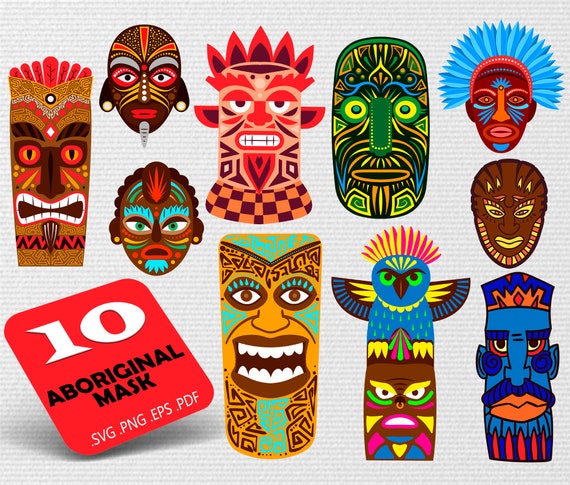The image is a vibrant, multi-colored digital collage of 10 distinct Aboriginal masks, set against a textured background with alternating blue and whitish vertical lines, creating a corrugated effect. The collage is arranged in a square format with no distinct border. In the bottom left corner, a red square contains the text "10 Aboriginal Masks, svg.png.eps.pdf" in white and black letters, indicating the available file formats of the images. The masks are diverse in design, featuring a broad spectrum of colors including reds, browns, blues, oranges, greens, and yellows. They vary in shape and style: some are long and narrow, resembling a tall popcorn box, while others are short and round, akin to an egg shape with elongated ears. A few masks display unique characteristics, such as one with a bird atop, another with a pineapple-like top, and several portraying exaggerated human features. Overall, this detailed and colorful collection showcases a wide array of artistic interpretations of tribal masks, blending elements of human and mythical figures.